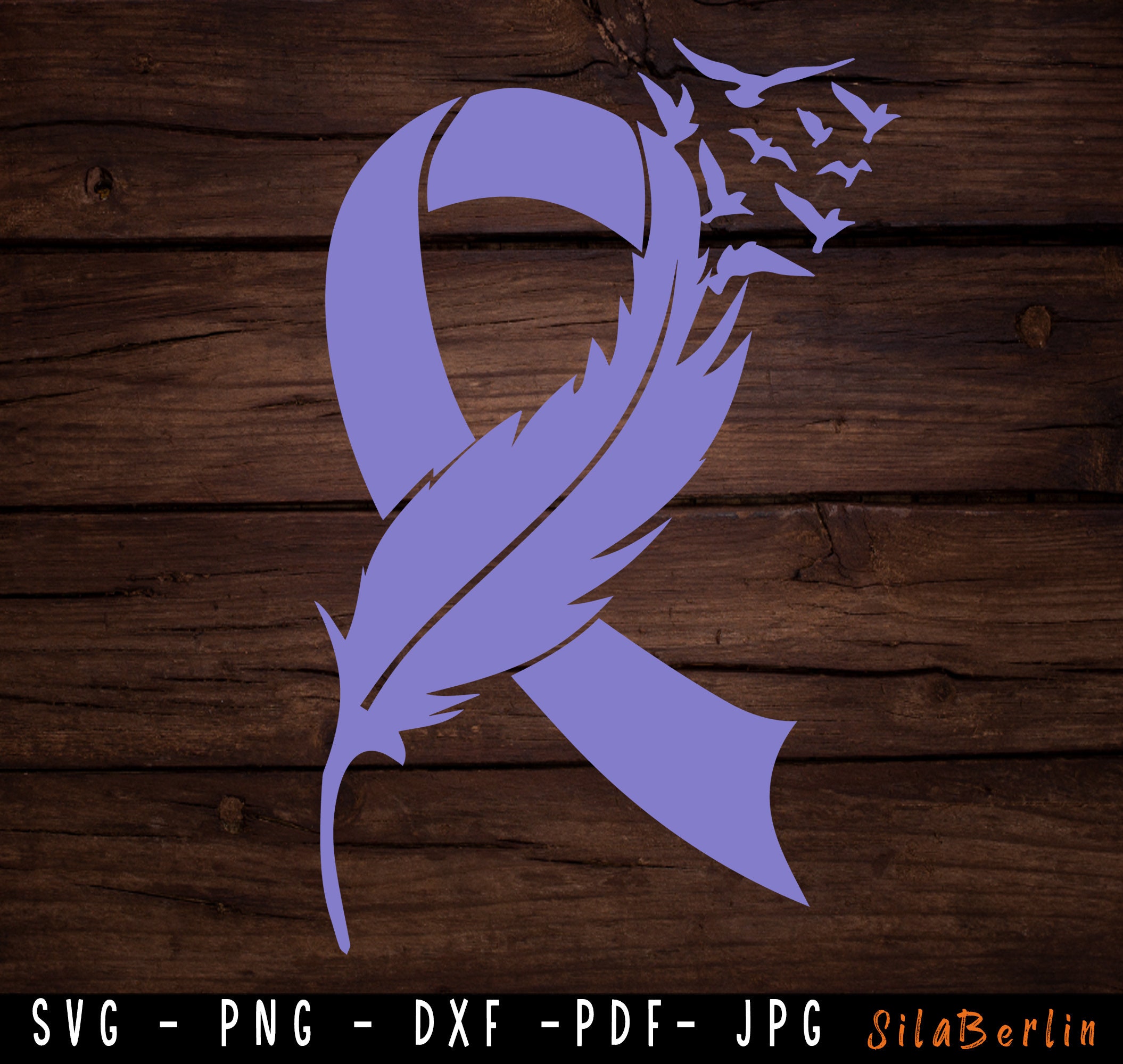This is a detailed digital illustration of a logo set against a wooden background. The logo takes the form of a periwinkle or light purple ribbon, reminiscent of an awareness ribbon. Unique to this design, the ribbon seamlessly transforms midway into a delicate feather on the left side, merging at the center-right. The feather's tip gives way to a flock of about 10 large birds, possibly geese, soaring upward and outward from the ribbon, symbolizing freedom or hope. At the bottom of the image, there is a black box listing various file formats: SVG, PNG, DXF, PDF, and JPG. Below this list, the name "CYLA BERLIN" appears in orange text.